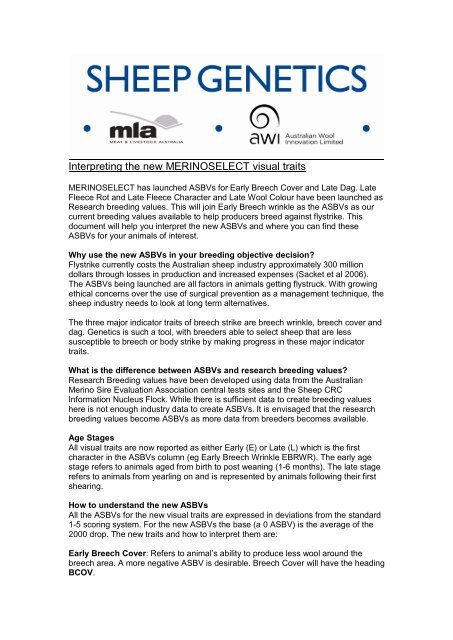This image depicts a detailed page on sheep genetics. The top of the page prominently features the title "SHEEP GENETICS" in a bold, navy blue all-caps font. Below the title, there are logos and names of two businesses: MLA and AWI (Australian Wool Innovation Limited). Both logos are separated by blue dots, with a grey checkmark and a spoon-like symbol above the MLA logo and a curly Q above the AWI initials in black. A horizontal line divides this header section from the rest of the content. The primary body of the page contains substantial text organized under several bold headlines, each introducing distinct segments of information. The main section starts with "Interpreting the New Merino Select Visual Traits" followed by various themed paragraphs with titles such as "Why Use the New ASBVs in Your Breeding Objective Decision?", "What is the Difference Between ASBVs and Research Breeding Values?", "Age Stages", "How to Understand ASBVs", and "Early Breech Cover". The document is printed on white paper with black text, providing comprehensive guidelines and details about sheep breeding and genetics.